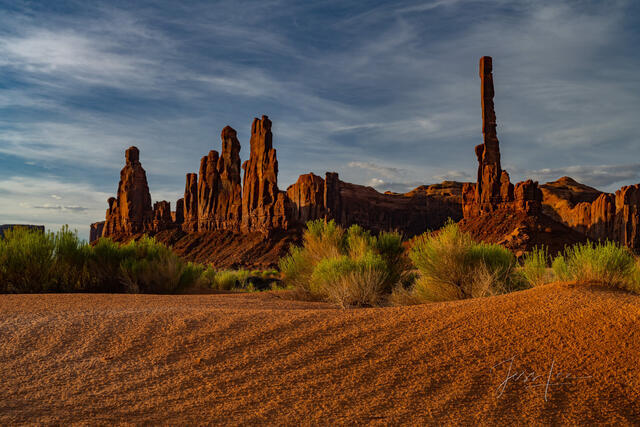This horizontally aligned rectangular photograph captures an outdoor scene at Monument Valley. The top portion of the image showcases a beautifully blended sky of clear blue and feathery white clouds. The sun appears low in the sky, casting a slight shadow over the scenery and contributing to a somewhat murky yet serene daylight atmosphere. 

In the middle ground, striking vertical stone columns and remnants of mesas and buttes dominate the landscape. These stone structures, which are varied in shape and size, are a medium to dark brownish color, possibly red-orange clay due to erosion. Some columns are intricately carved, resembling figures, while others appear more random and naturally formed. 

The foreground features patches of tall grass and small shrubberies with green tips and brownish bases sprouting from the sandy, rippled terrain. The sand, subject to wind action, appears similar to the formation of small dunes. 

Overall, the image vividly captures the unique interplay of natural elements, from the textured land and sculpted rock formations to the dynamic sky above.